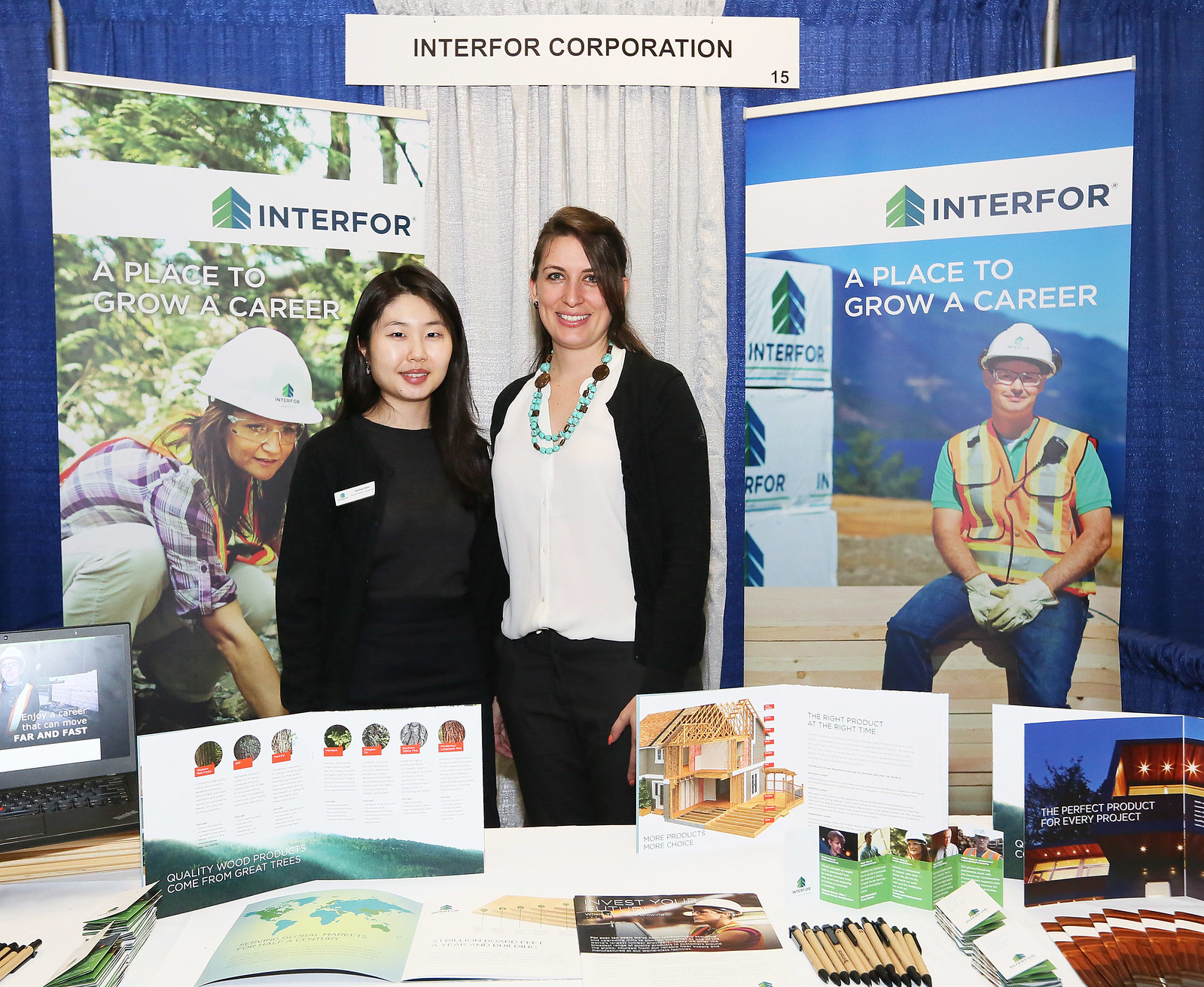In the photo taken at a job fair, two women are prominently posing at the center of their promotional booth for Interfor Corporation. They stand behind a table neatly arranged with various pamphlets, brochures, and a stack of pens, suggesting they are offering career information and giveaways. The woman on the left appears to be of Asian descent, with straight, dark black hair cascading past her shoulders. She wears a black blazer, a black blouse, and a white name tag, though the details on the name tag are not visible. Her lower half is obscured by the table's brochures. To her right stands a slightly taller Caucasian woman with long brown hair, partly obscured over one eye, and pulled back past her shoulders. She is dressed in a white button-up shirt, adorned with a statement teal necklace, and a black jacket and pants. 

The backdrop features a blue and white curtain flanked by two vertical banners displaying the Interfor Corporation logo. The banner on the left shows a woman in a high-visibility vest and hard hat kneeling in a forest, while the banner on the right depicts a person in a similar vest, helmet, and walkie-talkie, sitting on a pile of lumber with a scenic wooded area behind. Additionally, a central sign reads "Interfor Corporation" with the number "15" underneath. The table's arrangement, the corporate branding, and the professional appearance of the booth underscore the company's focus on career opportunities within the forestry and construction industries.